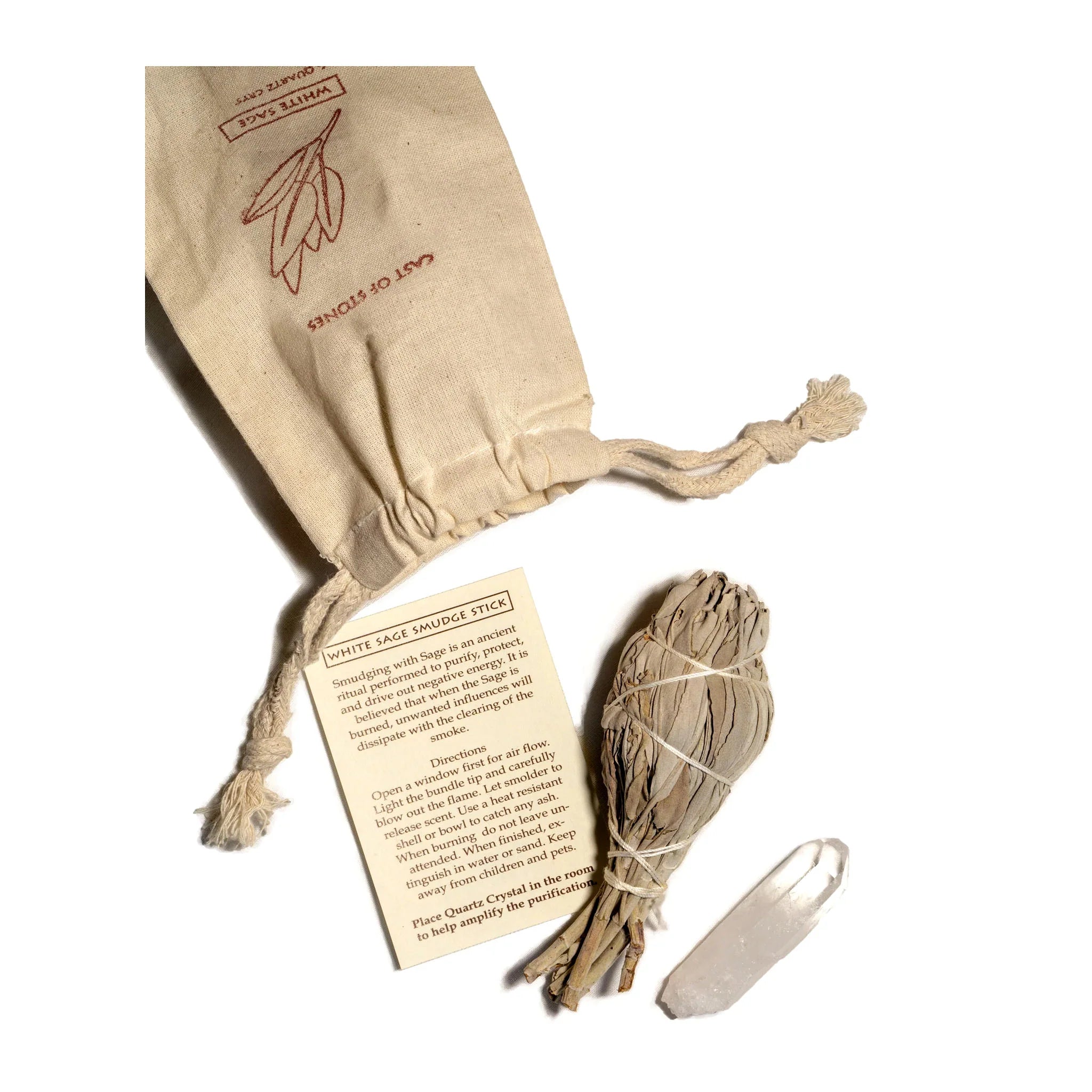In the image, against a white background, there is an assortment of items dominated by beige and brown hues. On the top left, an upside-down burlap sack marked with the text "cast of stones" is partially visible. The bag, detailed with tie strings, features an emblematic design of a leaf with the inscription "white sage" underneath it. Adjacent to the bag, a piece of paper provides detailed instructions and information, prominently displaying the heading "White Sage Smudge Stick." The text elaborates on the ancient ritual of smudging with sage to purify, protect, and drive out negative energy, and includes directions for safe usage. Beside these items lies a bundle of dried white sage leaves, carefully folded and tied together, meant to be used as a smudge stick. Additionally, a small stick and some materials resembling chalk can also be seen. This ensemble appears to form a kit for smudging, aiming to cleanse the surroundings and amplify the purification process with a quartz crystal.